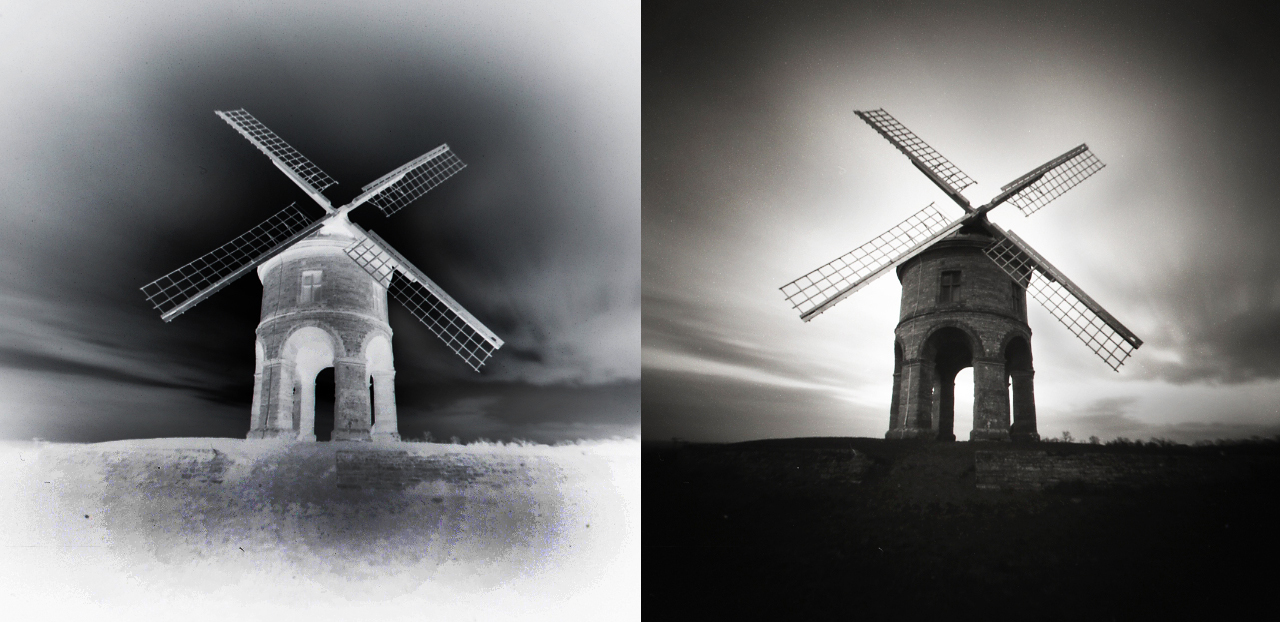The image comprises of two side-by-side black and white photographs of a stone windmill with a partially open base and a more enclosed upper portion resembling a building that might be inhabitable. The foreground includes a grassy field, and the structure is positioned centrally, rising prominently against a cloudy sky backdrop. The windmill features four large blades with grid-like patterns that resemble solar panels or netting, angled slightly from the roof. In each photograph, details differ slightly due to alternative exposures: The photo on the left is a negative image, causing the windmill and grass to appear bright, accentuating elements such as the tall arched doorways and windows on the windmill’s upper part, as well as clearly defined clouds. The right photo is a standard black and white exposure, giving the windmill a darker, more rugged look, with the sky taking on a late-sunset ambiance with deeper contrast between light and dark areas. The twin images, though identical in composition, highlight distinct visual elements and textures, providing a comprehensive and moody portrayal of this architectural structure.